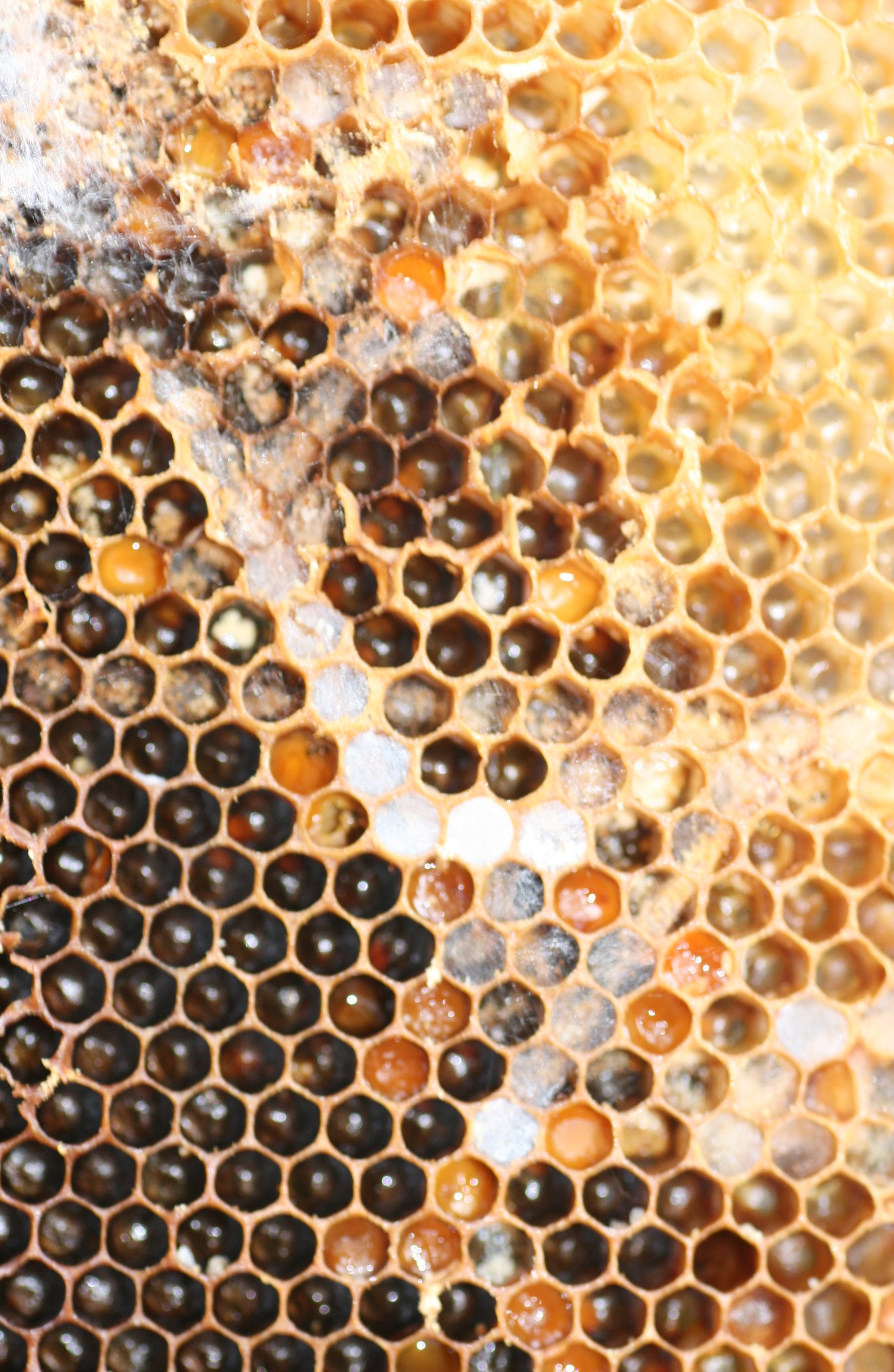This image is a slightly out-of-focus, close-up color photograph of a beehive's honeycomb. The macro shot reveals numerous symmetrical sections resembling bubbles, each in varying shades of brown, gold, bronze, and yellow. There is a rich texture and color variation throughout the honeycomb, with areas showing dark brown honey, light amber, and even pale yellow hues. A distinctive white streak runs from the top left corner at an angle, adding to the complex visual pattern. The photograph's lighting is flat, lending a muted overall tone, with some portions of the honeycomb appearing unfilled, particularly towards the bottom right. This highly detailed and zoomed-in image captures the intricate, messy beauty of the beehive structure.